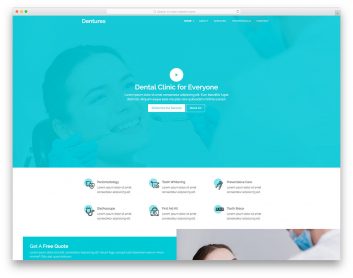The image shows a dental clinic advertisement designed with a clean and professional layout. At the center of the image, there is a prominent logo featuring a white dot encircling a blue dot, with the text "Dental Clinic for Everyone" displayed below it. Beneath this, there is a hyperlink button, with both white and background-colored variations.

The backdrop of the image is primarily light blue, with a subtle and slightly blurred image of a woman undergoing a dental check-up by a dentist on the right side. At the top of the advertisement, the brand name "UTC Dental" is faintly visible.

In the top right corner of the image, there is a widget area that appears to contain interface buttons or icons. Below this section, there are six descriptive icon sections arranged in two rows of three. Each icon section features a title in bold black text with a brief description in smaller gray text, all set against a white background that contrasts with the light blue surrounding it.

The bottom of the advertisement transitions into another light blue section, this time not fully extending to the left, leaving a white margin. On the bottom right, the light blue section contains white text inside a blue box, alongside a more defined image of the woman receiving dental care. This layout balances informative content with visual appeal, emphasizing the clinic's comprehensive dental services.